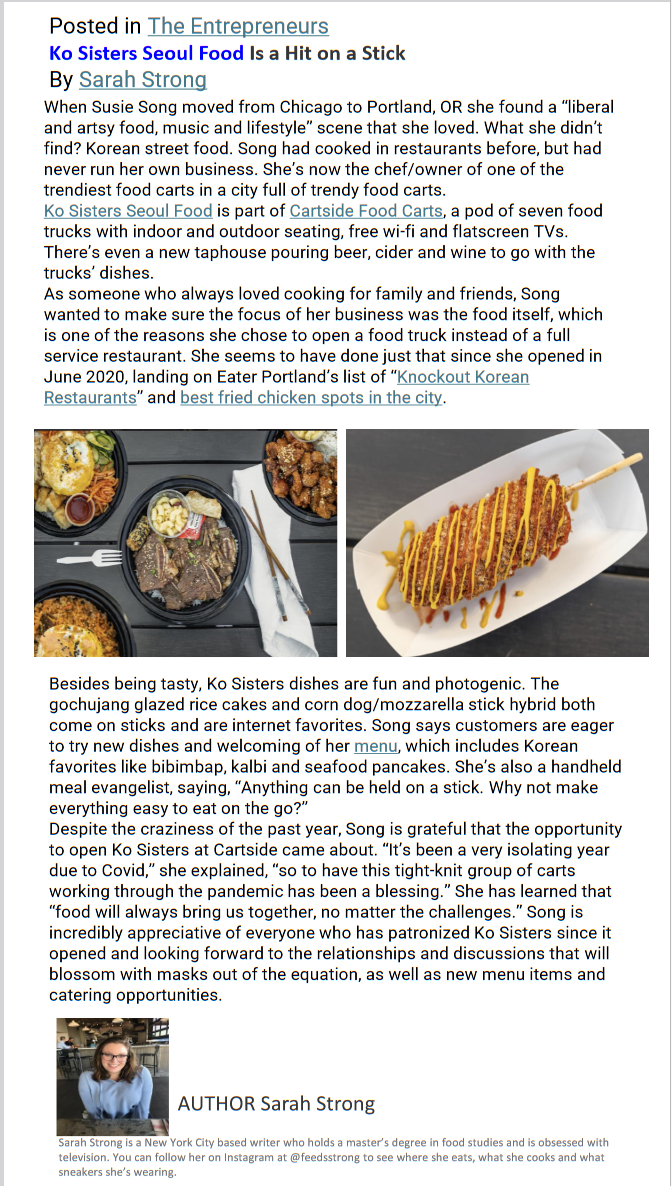**Caption:**

This image, captured from a cell phone screen, displays a post from a platform titled "Entrepreneurs." At the top, the screen displays "Entrepreneurs," followed by a headline "Co-Sisters Soul Food is a Hit on a Stick" authored by Sarah Strong.

The content begins with a detailed narrative about Susie Song, a chef who relocated from Chicago to Portland, Oregon. Despite embracing the vibrant, liberal, and artsy scene of Portland, Susie noticed a lack of Korean street food, an area she was passionate about. This led her to establish "Co-Sisters Soul Food," now one of the most popular food carts in a city renowned for its diverse array of food trucks.

Further description highlights that "Co-Sisters Soul Food" is part of "Cart Side Food Carts," a collective of seven food trucks offering indoor and outdoor seating, free Wi-Fi, and flat-screen TVs for customer entertainment. The location also features a newly opened tap house serving beer, cider, and wine, perfectly complementing the delectable dishes from the food trucks.

The post includes two images, followed by additional paragraphs elaborating on the stories and experiences related to the food cart. At the very end, the author's name, Sarah Strong, is reiterated, with fine print information available at the bottom of the screen.